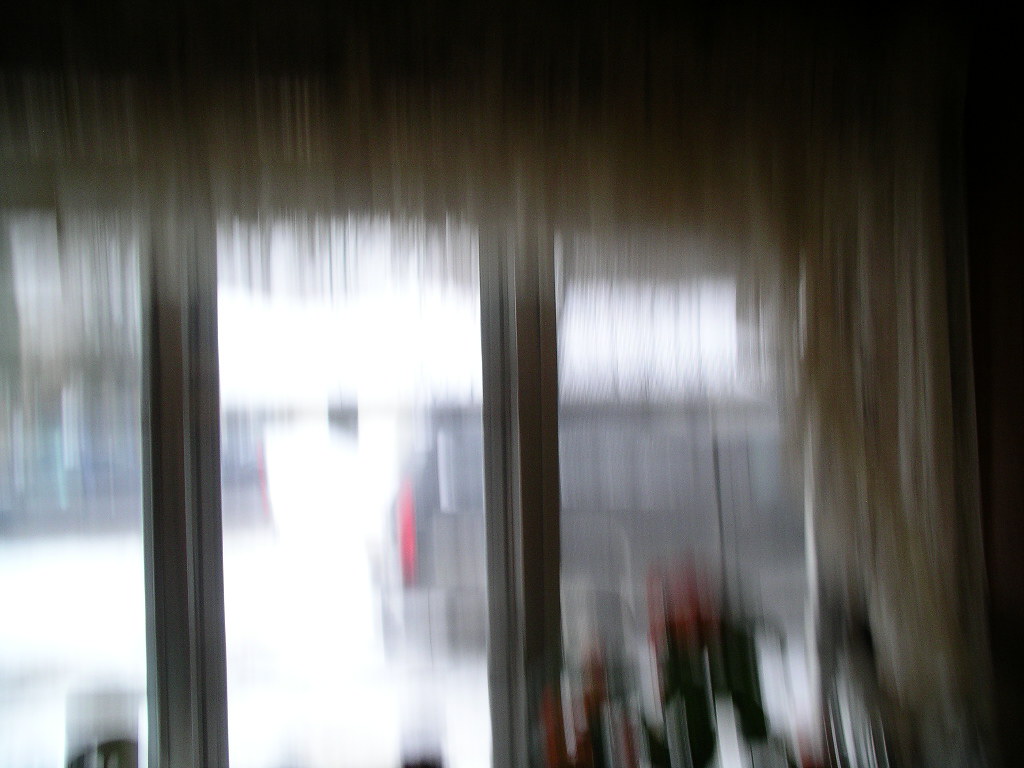The image, though blurry, captures a scene featuring three windows adorned with sheer curtains. Beyond the translucent fabric, the outline of a pickup truck is discernible, accentuated by a solitary red taillight. The rightmost window is further embellished with a set of longer drapes cascading down the side. Inside the room, positioned in front of the right window, there are objects that resemble plants, housed in black bases topped with small red accents. Additionally, the scene includes what appear to be candles: a smaller one situated in the middle window and a larger one gracing the left window.